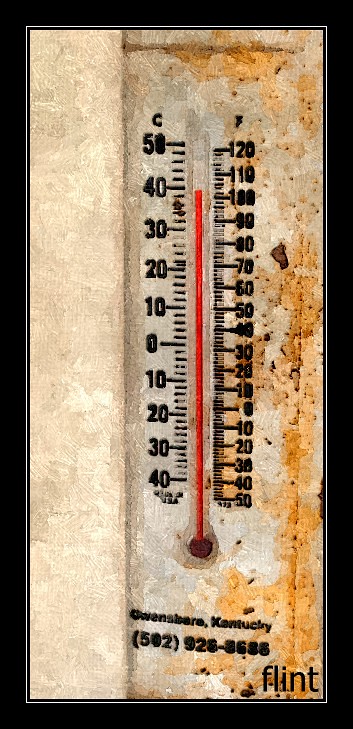The portrait-oriented image features a built-in wall thermometer, prominently positioned against a yellowing and decaying wall. The thermometer, which shows temperature readings in both Fahrenheit (on the right) and Celsius (on the left), includes a visible tube filled with red liquid that rises and falls with temperature changes. The temperature markings are inscribed directly onto the wall in thick black ink. The right side of the wall, especially near the thermometer, shows significant signs of decay. Just below the thermometer, text is visible on the wall, stating "Owensboro, Kentucky," followed by a phone number: 502-926-8688. This text is printed in very thick lettering, making it somewhat difficult to discern clearly. In the bottom right corner of the image, a logo is present. A thin black border with a white line frames the entirety of the image.